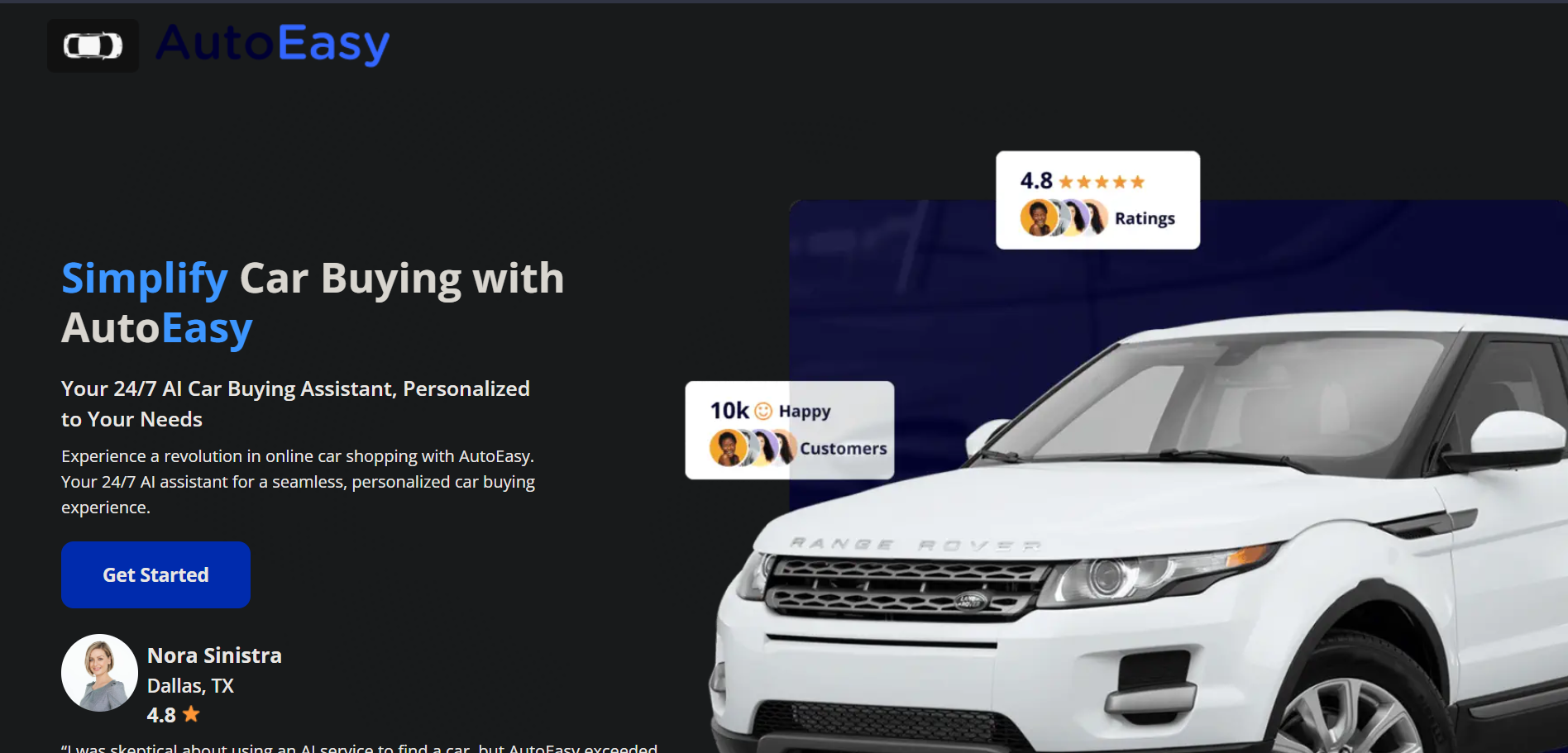The image is a screenshot of a website dedicated to car shopping. In the top left corner, the word "Auto" appears in a dark font that blends into the background, partially obscured, making the bright blue "easy" stand out prominently next to it. Below this, a tagline reads "Simplify car buying with Auto Easy" in a combination of blue and white font, emphasizing the ease of use. The text further elaborates: "This is your 24/7 AI car buying assistant personalized to your needs. Experience a revolution in online car shopping with Auto Easy, the 24/7 AI assistant for a seamless, personalized car buying experience." A "Get Started" button is displayed in blue with white font.

To the left beneath this main text, there is the name "Nora Sinatra, Dallas, Texas," accompanied by a 4.8-star rating. On the right side of the image, there is a top-down view of a white car, positioned as if seen from the driver's side front, against a dark blue background that fades before reaching the top of the page. Additionally, two rating indicators display customer satisfaction: one shows "4.8 Gold Stars" and another notes "10K Happy Customers," both within white rectangles with black writing. Iconic symbols for users are represented by black and blue circles.